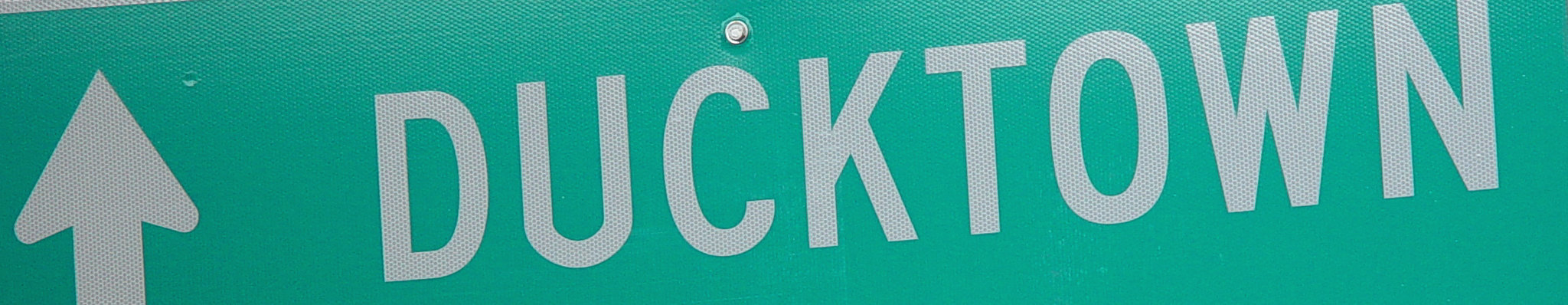This photograph features a rectangular street sign cropped against a plain white background, omitting any visible frame. The sign itself is green with white text and details. On the left side of the sign, an arrow originates from the bottom left corner, pointing upwards. Adjacent to the arrow, the word "DUCKTOWN" is presented in capital letters, arranged slightly diagonally with a tilt: the letter "D" is lower while the concluding "N" sits higher. Positioned immediately above the letter "C," a small bolt secures the sign. Additionally, the top right portion of the final letter "N" is truncated. A slim white border is visible at the upper left corner of the sign, adding contrast.